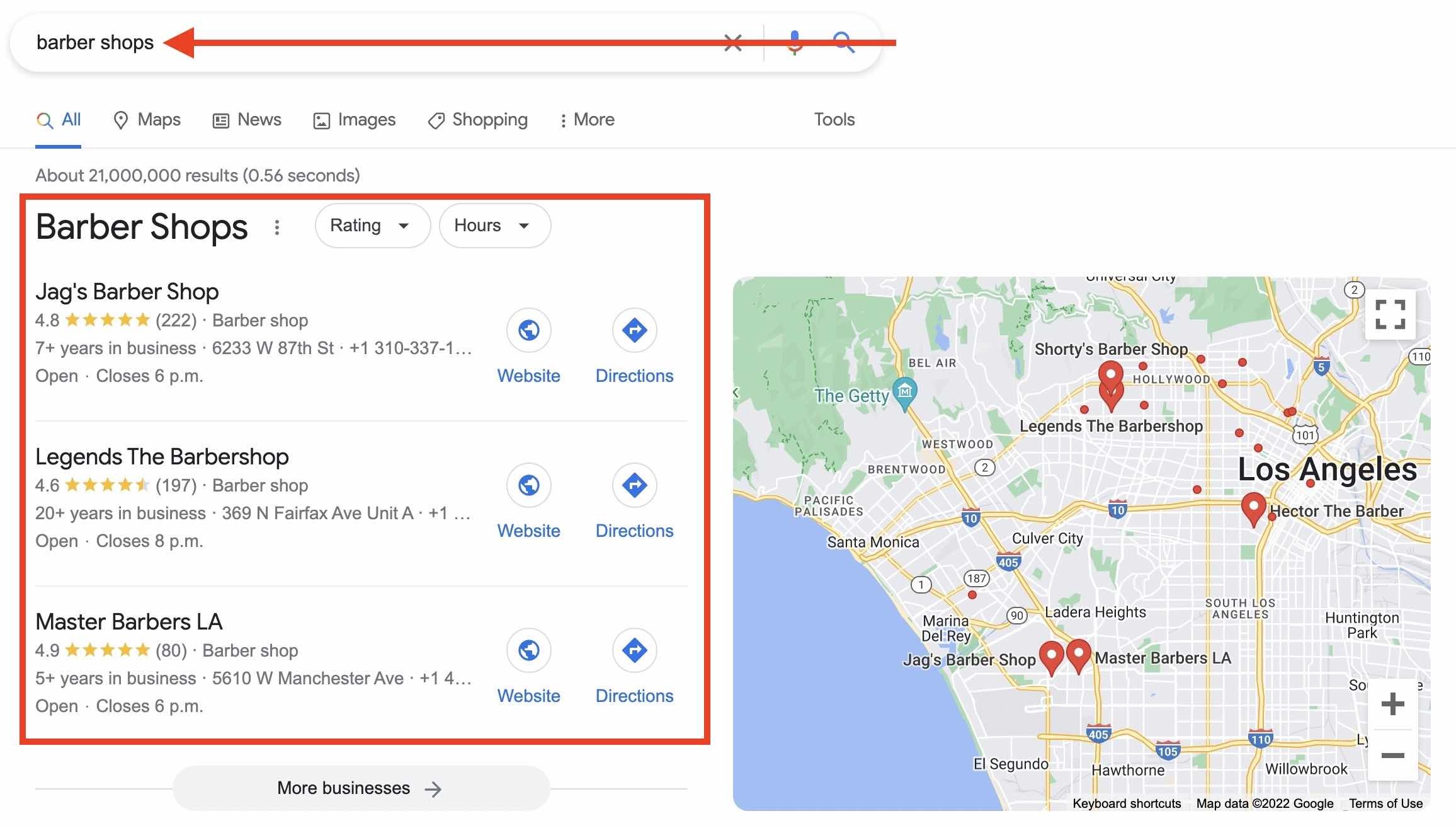A Google search results screenshot is depicted for the query "barbershops." The search bar is prominently displayed at the top of the image, with an arrow running through it, pointing directly at the section below. 

Below the search bar, there's a menu with options: All, Maps, News, Images, Shopping, and More. The "All" option is selected, revealing approximately 21 million results found in 0.56 seconds. In a red-highlighted box, the term "barbershop" appears alongside dropdown menus for ratings and hours.

The top search result is Jag's Barbershop, which boasts a rating of 4.8 stars and over 7 years in business. The listing includes the barbershop's address, hours of operation, and links for the website and directions. The second result is Legends the Barbershop, rated 4.6 stars, also accompanied by links for the website and directions. The third result features Master Barbers LA, with an impressive rating of 4.9 stars. Below these results, there's a button labeled "More businesses," accompanied by a right-pointing arrow.

On the right side of the search results, a map of West Los Angeles is shown. Several barbershops, including the ones listed, are marked with red location markers, indicating their positions. The close-up view provides a clear layout of their geographic distribution within the area.